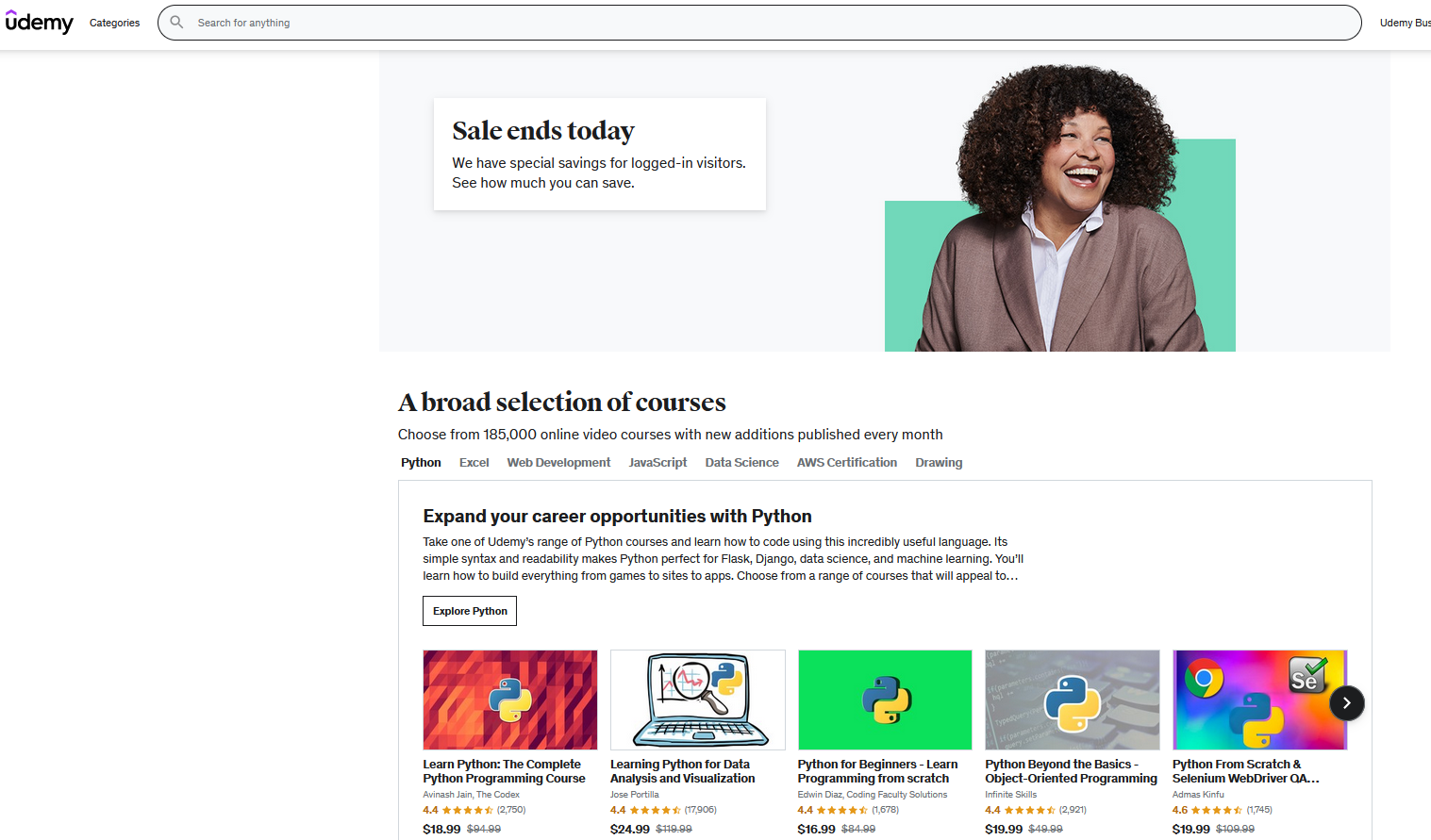This image is a highly detailed screenshot of a webpage viewed in landscape mode, showcasing various elements of an online learning platform. 

In the upper left corner, the U-D-E-M-Y logo is prominently displayed, followed by a "Categories" link. Adjacent to this is a search bar with the placeholder text "Search for anything." Moving to the upper right, the partially visible text "U-D-E-M-Y-B-U-S" indicates additional navigation options, possibly "Udemy Business," though the text is cut off.

The content area begins with an urgent call to action: "Sale ends today. We have special savings for logged-in visitors. See how much you can save." To the right of this message, a slightly dark-skinned woman with voluminous, curly hair is depicted, wearing a white button-up top and a brown jacket.

The next section emphasizes the vast array of courses available on the platform: "A broad selection of courses: Students choose from 185,000 online video courses with new additions published every month." Specific courses are highlighted, including Python, Excel, web development, JavaScript, data science, AWS certification, and drawing. The focus is on Python, underscored by a themed section that reads: "Expand your career opportunities with Python. Take one of Udemy’s range of Python courses and learn how to code using this incredibly useful language. Its simple syntax and readability make Python perfect for Flask, Django, data science, and machine learning."

Beneath this informative text, there is a prominent button labeled "Explore Python," inviting users to delve deeper into the Python course offerings.